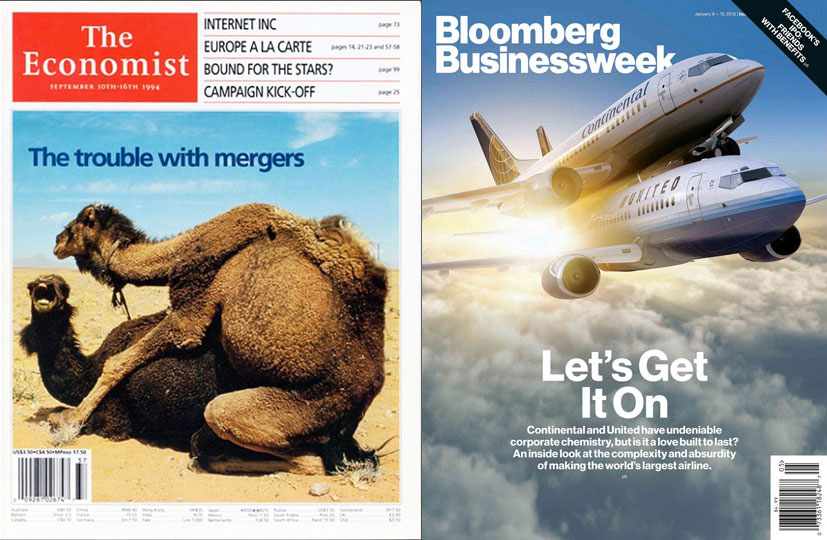This digital image showcases the covers of two prominent magazines. 

**Left Magazine - The Economist (September 10th-16th, 1994)**: The cover portrays a satirical illustration featuring two camels in a desert landscape filled with sand. One camel is mounted on top of the other, with the lower camel's mouth open as if reacting to the situation. Above the camels, the headline reads "The Trouble with Mergers," perhaps indicating the challenges and complications often associated with corporate mergers. Other headlines on the cover include "Internet Incorporated," "Europe a la carte," "Bound for the Stars," and "Campaign Pick Off."

**Right Magazine - Bloomberg Businessweek**: This cover features a visual of two large commercial airplanes, specifically from Continental and United Airlines. The illustration shows one airplane positioned above the other, visually reinforcing a theme of corporate mergers or competition within the airline industry.

The juxtaposition of these covers highlights thematic elements of business, mergers, and corporate dynamics.